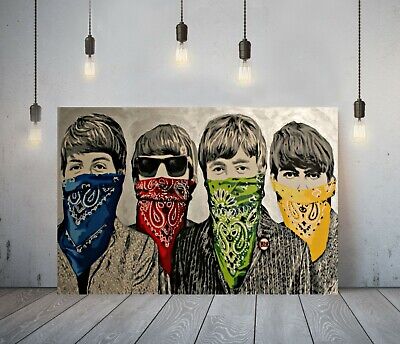The image depicts a black and off-white painting of The Beatles, showcasing Paul McCartney, Ringo Starr, John Lennon, and George Harrison each wearing distinctive bandanas over their noses and mouths. Paul stands on the far left with a blue and white bandana, followed by Ringo with a red and white bandana, John with a green and white bandana, and George with a yellow and black bandana. The painting leans against an off-white wall above a gray planked wooden floor in what appears to be an art gallery. Six Edison-style light bulbs hang from the ceiling at varying heights, illuminating the artwork with a soft glow.